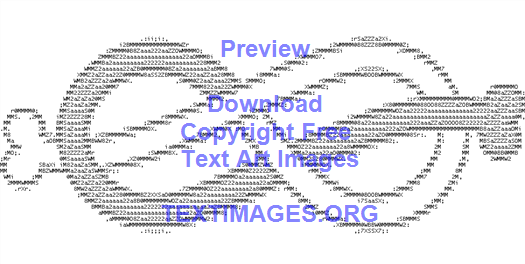This horizontal, rectangular, borderless image features a detailed computer-generated ASCII art drawing of a rope tied into an intricate knot. The knot forms a complex pattern, resembling two interlocking loops—one with dark lines and the other with lighter, white lines—creating an illusion akin to an infinity symbol. The entirety of the artwork, rendered with straight lines, numbers, and typewriter fonts, appears like a sketch or an abstract pretzel morphing into bones at both ends. Superimposed over this monochromatic ASCII art is a series of blue texts arranged vertically: "Preview," "Download," "Copyright-Free Text Art Images," and prominently at the bottom, "TextImages.org." The image suggests that by visiting TextImages.org, one can freely download similar text-based images for use in advertising or other creative projects.